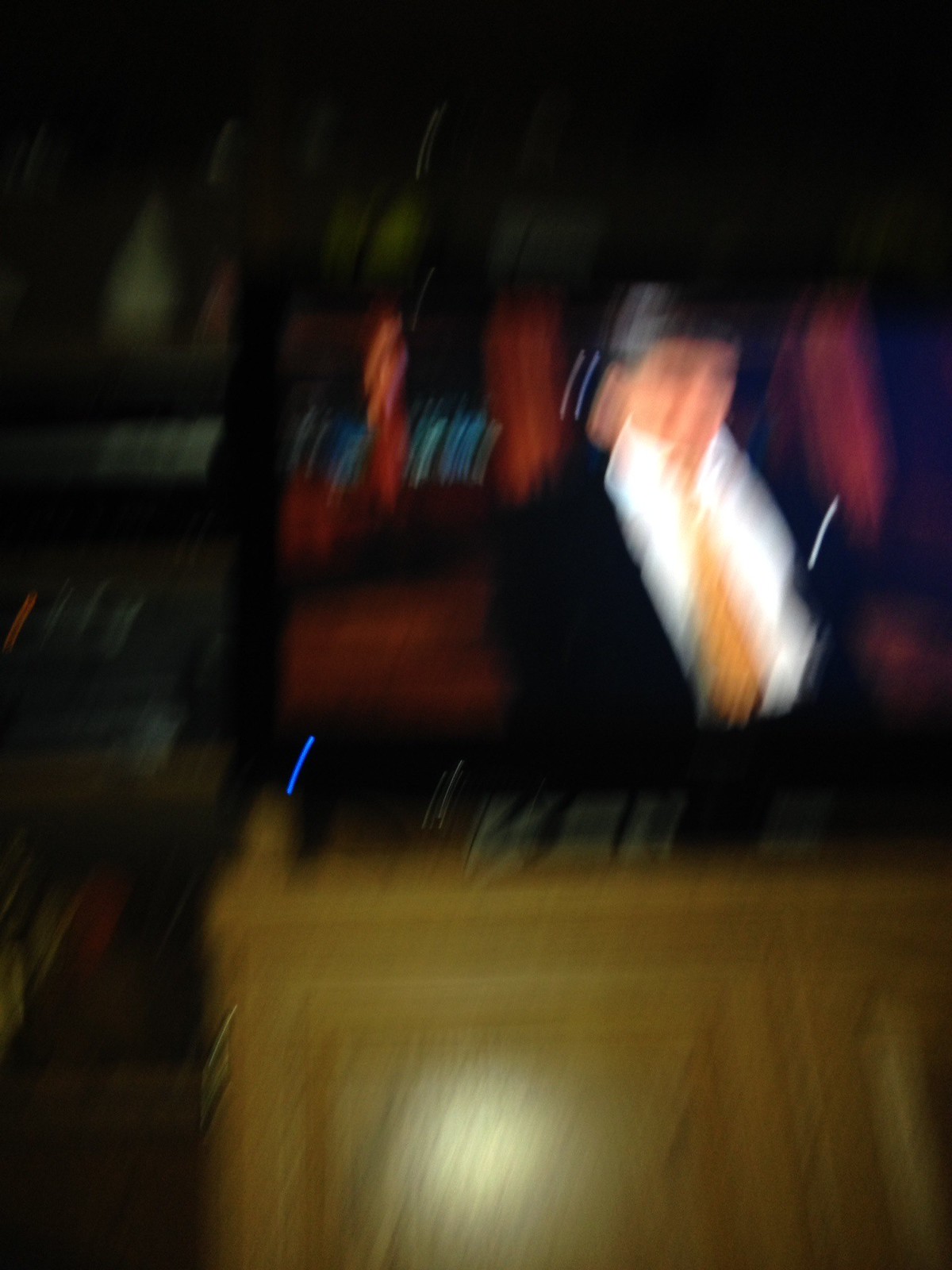This photograph captures a cozy living space featuring a light tan-colored wood cabinet with a flat top and two front doors. The cabinet's doors are fitted with visible metal hinges, although the image doesn't show the door handles. A bright spot of light is reflecting off the front of the cabinet, adding a touch of luminescence. Atop the cabinet sits a sleek black television with a thin, one-to-two inch black border around the screen. A small, bright blue dot in the bottom corner indicates that the television is powered on. Displayed on the TV is the image of a man dressed in a black suit jacket, a white shirt, and an orange tie, standing in a room with reddish-colored walls. The television image appears slightly blurred, making it difficult to discern more detailed features.